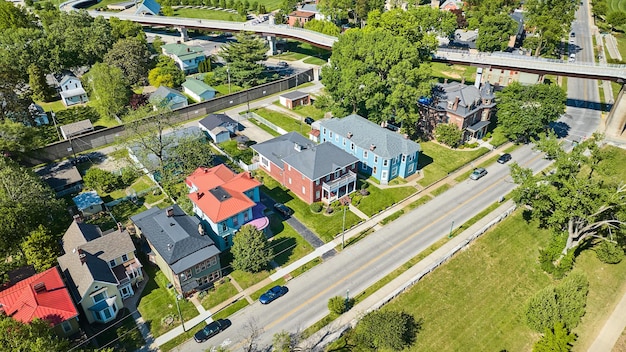This detailed overhead shot, likely taken by a drone, captures a picturesque neighborhood bathed in sunlight. A gray asphalt street with a yellow stripe runs horizontally through the scene, separating a lush, well-manicured field of grass from a line of six distinct homes. These residential houses, featuring vibrant rooftops in shades of red, gray, gunmetal gray, and dark blue, are lined up along the road. The left side of the street has two parked vehicles, mirrored by another two on the right. No cars are seen driving on this quiet street.

In the foreground, a raised bridge or overpass elevates above the serene neighborhood, adding a dynamic layer to the scene. Each house is accompanied by neatly trimmed front and backyards dotted with trees. Fences delineate the properties, behind which additional sheds and more homes can be spotted, further showcasing the orderly layout of this well-maintained area. The bright sunlight highlights the vivid colors and lush greenery, portraying a peaceful, vibrant community in the midst of a clear, sunny day.